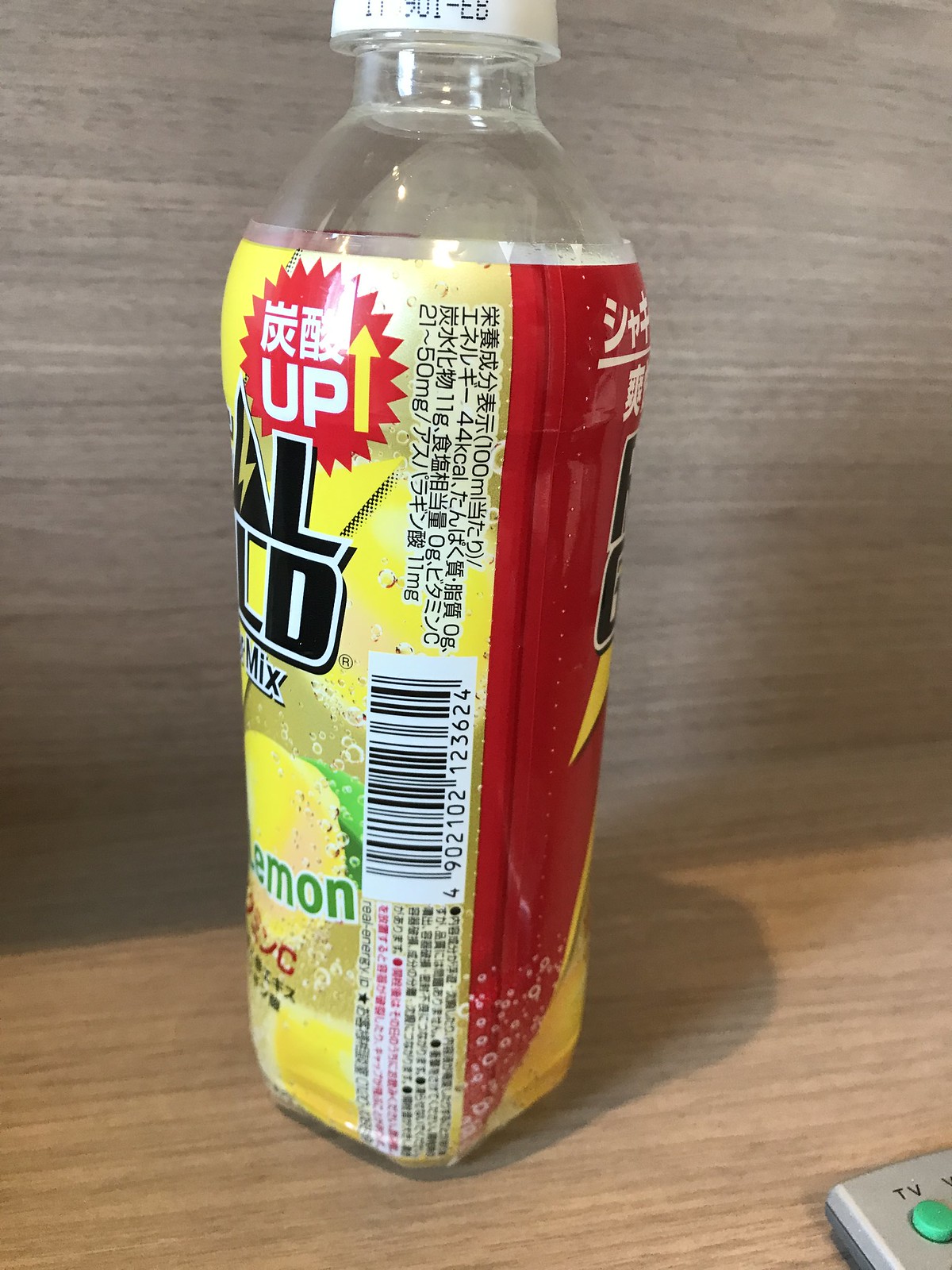This photograph captures a plastic bottled drink resting on a wooden shelf. The bottle features a white cap and a label that wraps around it, positioned sideways in the image. The label is predominantly yellow on the left side and red on the right side. 

In the center of the label, there is a barcode flanked by Asian writing. The left side of the label, which is yellow, showcases the word "lemon" and an illustration of a lemon with bubbles. A red, medallion-like design is situated at the top of the yellow section, featuring white font that reads "UP" alongside a yellow upward-pointing arrow and additional Asian writing.

The red portion of the label displays rising bubbles, enhancing the refreshing theme of the beverage. The flavors suggest a lemon variety. Finally, in the bottom right corner of the photo, there is a partial view of a remote control, adding context to the setting.